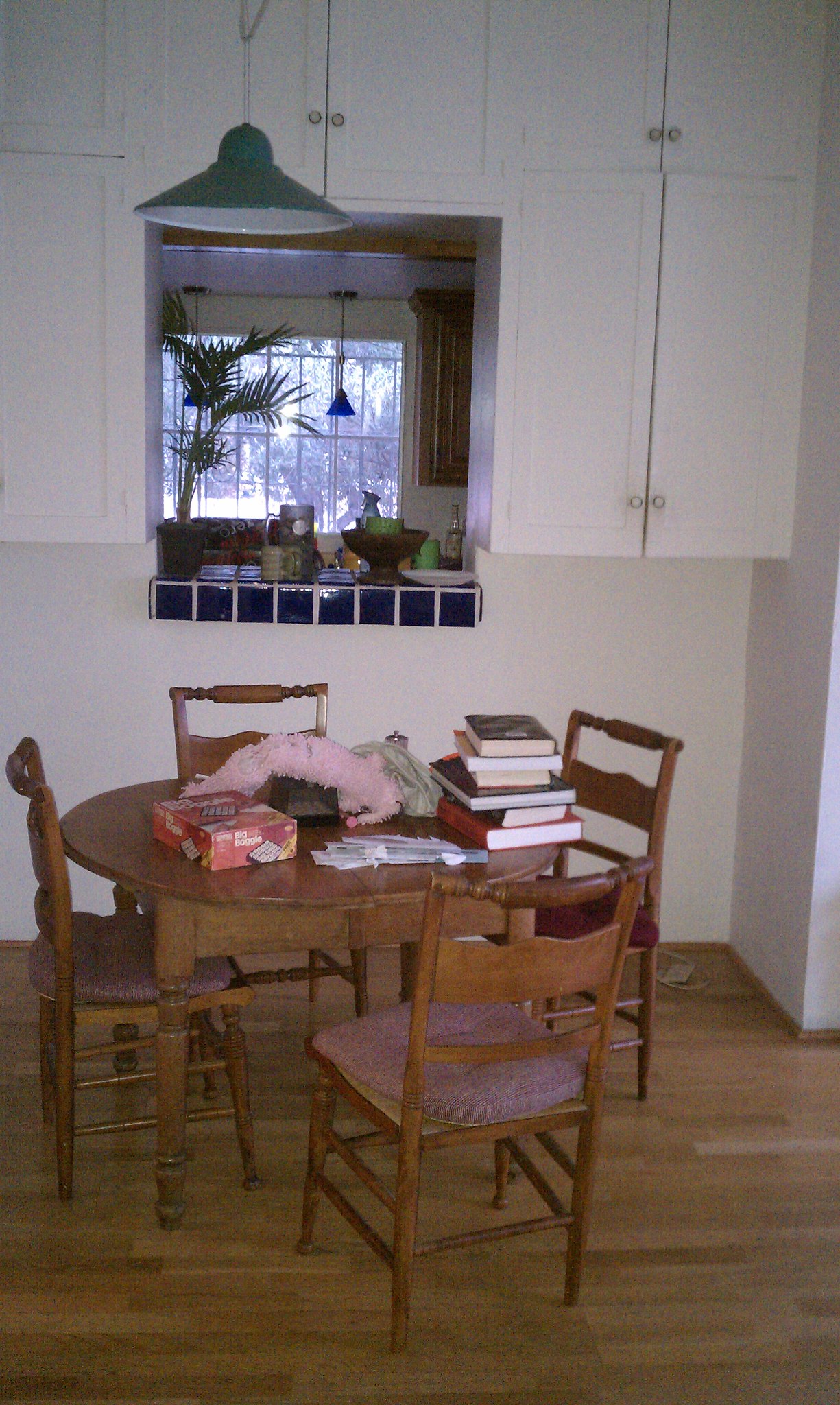The image portrays a cozy kitchen scene captured in a vertical rectangular format. In the background, white cabinets with detailed paneling and small silver circle knobs are prominently featured. A square cut-out section in the center of the cabinets offers a glimpse into the adjacent kitchen area, where brown, ornately framed cabinets are visible. Through a window composed of numerous small rectangular panes, daylight filters in, highlighting the greenery of trees outside.

On the kitchen counter, situated within the cut-out section, there is a plant, set against a backdrop of blue tiled squares. The countertop also hosts a fruit bowl and a variety of knickknacks. Appealing blue pendant lights hang from the ceiling, adding a touch of character to the space.

The room's floor is composed of thin, brown wooden planks that suggest an older, classic style. The white walls complement the overall aesthetic. In the center of the room, a circular brown wooden table, accompanied by four seemingly aged chairs, serves as a focal point. The table is cluttered with everyday items: a stack of books, what appears to be a game, a pink object, and a pile of mail, reflecting the casual nature of a well-lived-in space.